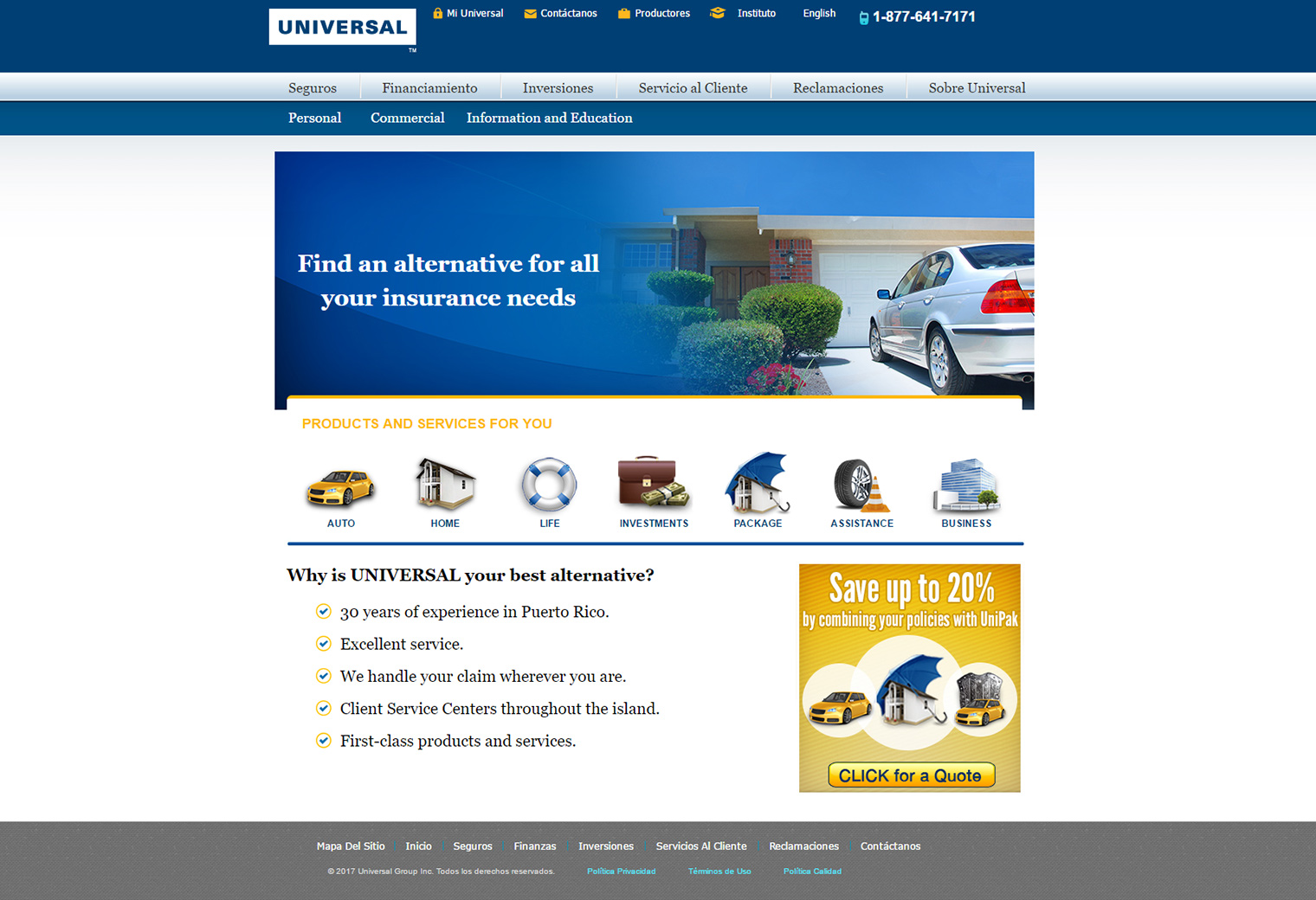**Screenshot of the Universal Insurance Company's Website - Bilingual Interface**

This image depicts a screenshot from the website of Universal Insurance Company, which primarily operates in Puerto Rico. The website offers bilingual support, allowing users to choose between Spanish and English, with the default language set to Spanish. Prominently displayed is the company's tagline, "Find an alternative for all your insurance needs." 

A visible section of the website includes a customer service phone number: 1-877-641-7171. The site organizes its offerings into several categories: Personal Insurance, Commercial Insurance, as well as Information and Education about various insurance products.

The insurance options include various types, such as Auto, Home, Life, Investment, Package, Assistance, and Business Insurance. Icons representing each category facilitate easy navigation for users.

Highlighted on the page is a section titled "Why is Universal your best alternative?" This part emphasizes several key points:
- Over 30 years of experience in Puerto Rico.
- Excellent service.
- Capability to handle claims wherever the client goes.
- Client service centers throughout the island.
- First-class products and services.
Additionally, there is a promotional box that advertises, "Save up to 20% by combining your policies with Unipack," along with an invitation to "Click for a quote."

This comprehensive layout reflects Universal Insurance Company's commitment to providing extensive support and quality services to its clients.